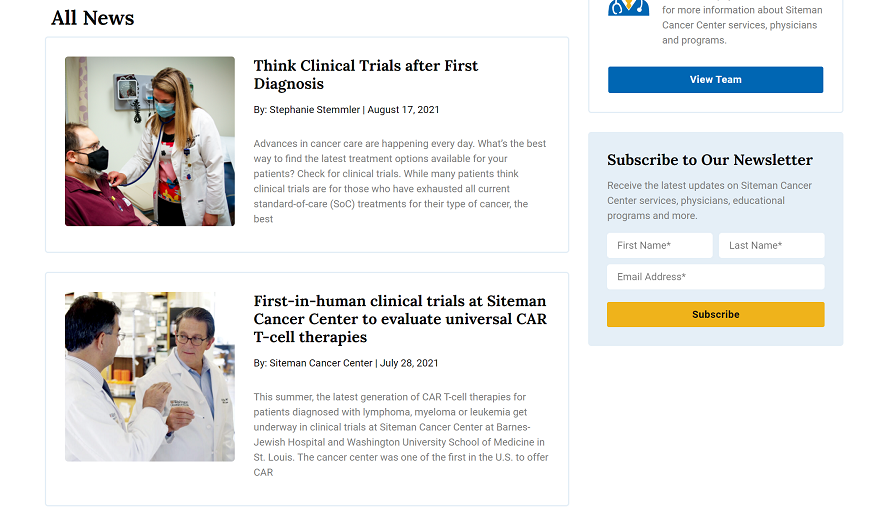**Caption:**

"Advances in cancer care are happening every day. On August 17, 2021, Stephanie Bamler reported on the importance of clinical trials following a cancer diagnosis. The most effective way to find the latest treatment options for patients is to explore ongoing clinical trials.

At Sightman Cancer Center, a pioneer in offering CAR T-cell therapies, significant strides are being made. On July 28, 2021, the center launched new first-in-human clinical trials to evaluate universal CAR T-cell therapies for patients with lymphoma, melanoma, or leukemia. This groundbreaking research is taking place at Barnes Jewish Hospital and Washington University School of Medicine in St. Louis.

For more information about Sightman Cancer Center's services, physicians, and programs, subscribe to their newsletter. Stay informed about the latest updates in cancer care by providing your first and last name along with your email address."